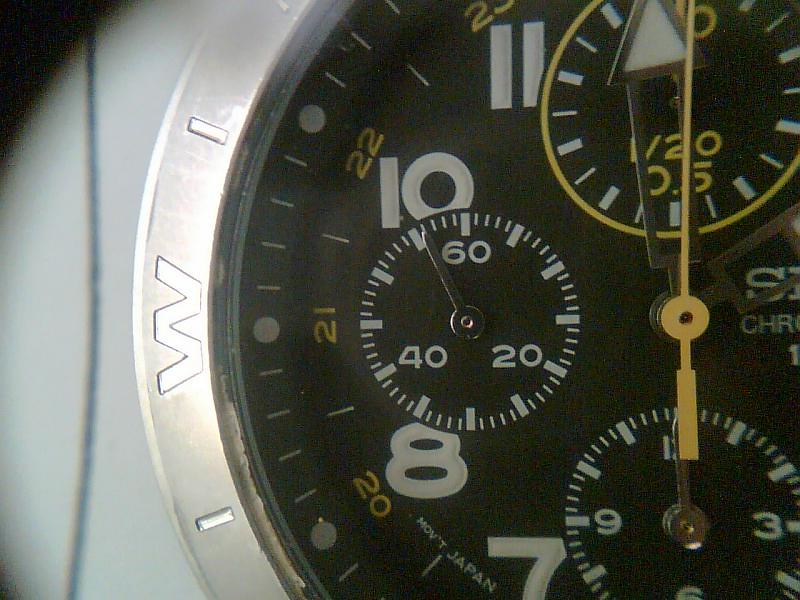This detailed close-up image captures the face of a round clock with intriguing precision. The primary clock face is black, adorned with bold white numbers marking the hours, specifically showcasing the numbers 7, 8, 10, and 11 prominently. The number 9 is notably obscured by a smaller inner clock dial that tracks seconds, indicated by white marks at 20, 40, and 60, with a solitary, slender hand extending from the center of this sub-dial. Additionally, diminutive yellow numbers, ranging from 20 to 23, ascend the clock face, adding a layer of complexity to its design.

Encircling the clock is a sleek silver frame, approximately half an inch in width, which features an engraved 'W' adding a touch of elegance. The background of the image reveals a white panel wall, providing a stark contrast that enhances the clock's intricate details.